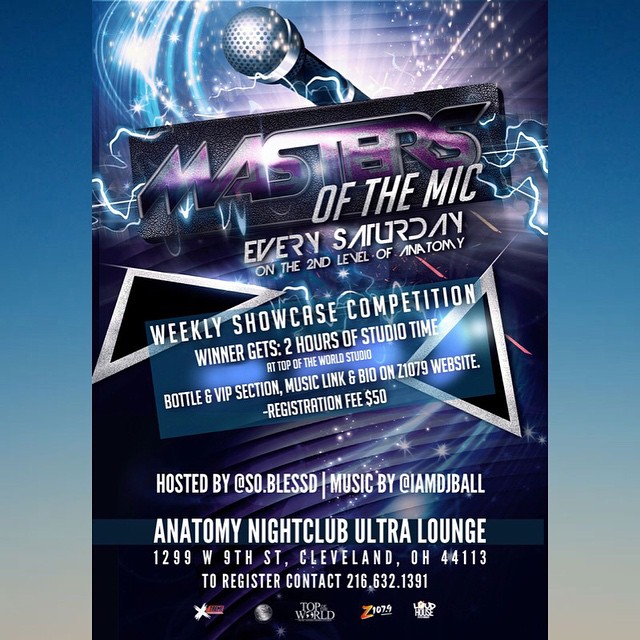The vibrant poster advertises an event at a nightclub, featuring a prominent microphone at the top center pointing to the upper left. The microphone has a black base and a silver platinum top. Above the microphone, electricity and sparks create a dynamic effect, with lightning-like charges emerging from the text, enhancing the dramatic visual. The centerpiece text reads "Masters of the Mic," with "Masters" in large, reflective purple font, and "of the mic" in white font. Beneath this, in white font, it announces that the event is held "Every Saturday on the Second Level of Anatomy."

The middle section of the poster declares the event as a "Weekly Showcase Competition," with the winner receiving "Two Hours of Studio Time at Top of the World Studio." Additional incentives include a bottle and VIP section, detailed information and music links on the Z1079 website, and a registration fee of $50.

At the bottom, more text specifies that the event is "Hosted by At.so.Blessed" and features music by "@IamDJBall." Further down, the venue is listed as "Anatomy Nightclub Ultra Lounge, 1299 W 9th Street, Cleveland, Ohio 44113." The contact number for registration is provided: 216-632-1391. 

The background of the poster features a mix of blue and purple hues, adorned with generic graphic elements such as silver triangles, swooshes of light, and sparks, adding to the visual chaos. The borders transition from dark blue at the top to gray at the bottom. At the bottom of the image, five small logos include symbols and text, among which "Top of the World" and "Z107.9" are discernible.